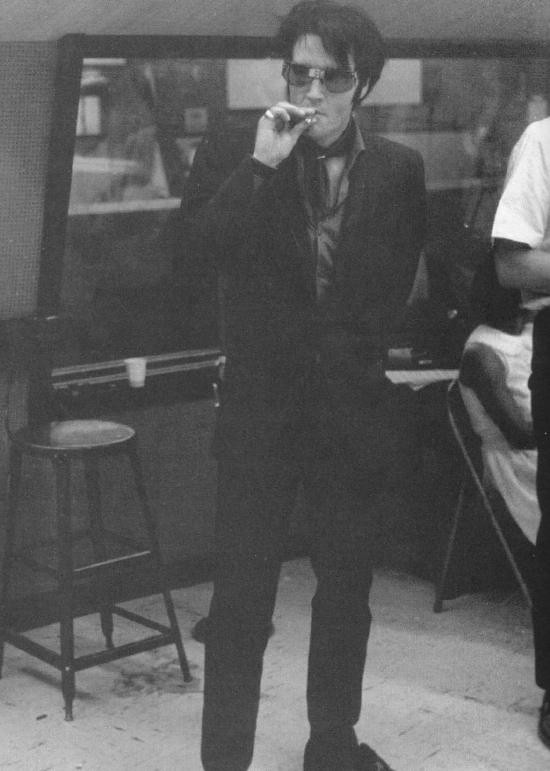This vintage image captures the legendary Elvis Presley in a candid moment. He is depicted smoking, possibly in a bar or recording studio, with a large mirror behind him that reflects the activities in the room. Elvis is dressed in a dark suit complemented by a dress shirt, a scarf, and dark pants with matching dark shoes. He wears his iconic glasses, which have a noticeable bridge between the lenses. To his right, a woman in a white dress is seated, and to his left, a man, also sporting a recognizable hairstyle and sunglasses, sits clad in a white shirt and dark pants. A stool is positioned behind Elvis, suggesting he may have been sitting there moments before. The setting is lively with a sense of camaraderie and a hint of mystique surrounding the King of Rock 'n' Roll.